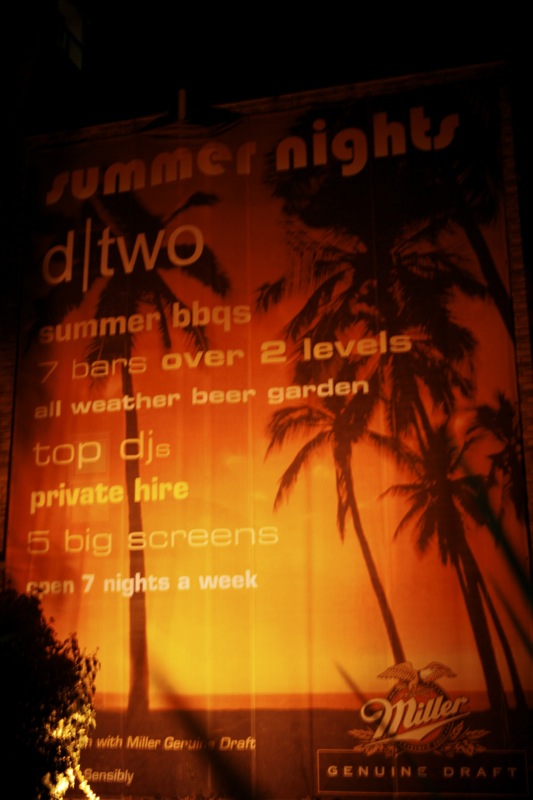The image features a nighttime banner or poster with a vibrant backdrop of a beach at sunset, emphasizing a warm, orange glow filling the sky and the sea as the sun dips below the horizon. Palm trees are silhouetted against the sunset, with one prominent tree on the left and several smaller ones on the right. The sign's edges darken into a brownish-black hue, enhancing the central glowing effect. 

At the top of the banner, in faint orange-brown letters, the words "Summer Nights" are displayed. Below it, a partially obscured line includes "D/T-W-O," possibly a date or code. The next lines detail various attractions in yellowish-orange letters: "Summer BBQ," "Seven bars over two levels," "All-weather beer garden," "Top DJs," "Private hire," and "Five big screens." Further down, in white letters, it announces "Open seven nights a week."

In the lower right-hand corner, the logo of Miller Genuine Draft is prominently featured, along with a small bush slightly visible nearby. The overall composition and details suggest this is an announcement for a summer event at a beach-side establishment, prominently advertising the amenities and activities available throughout the week.